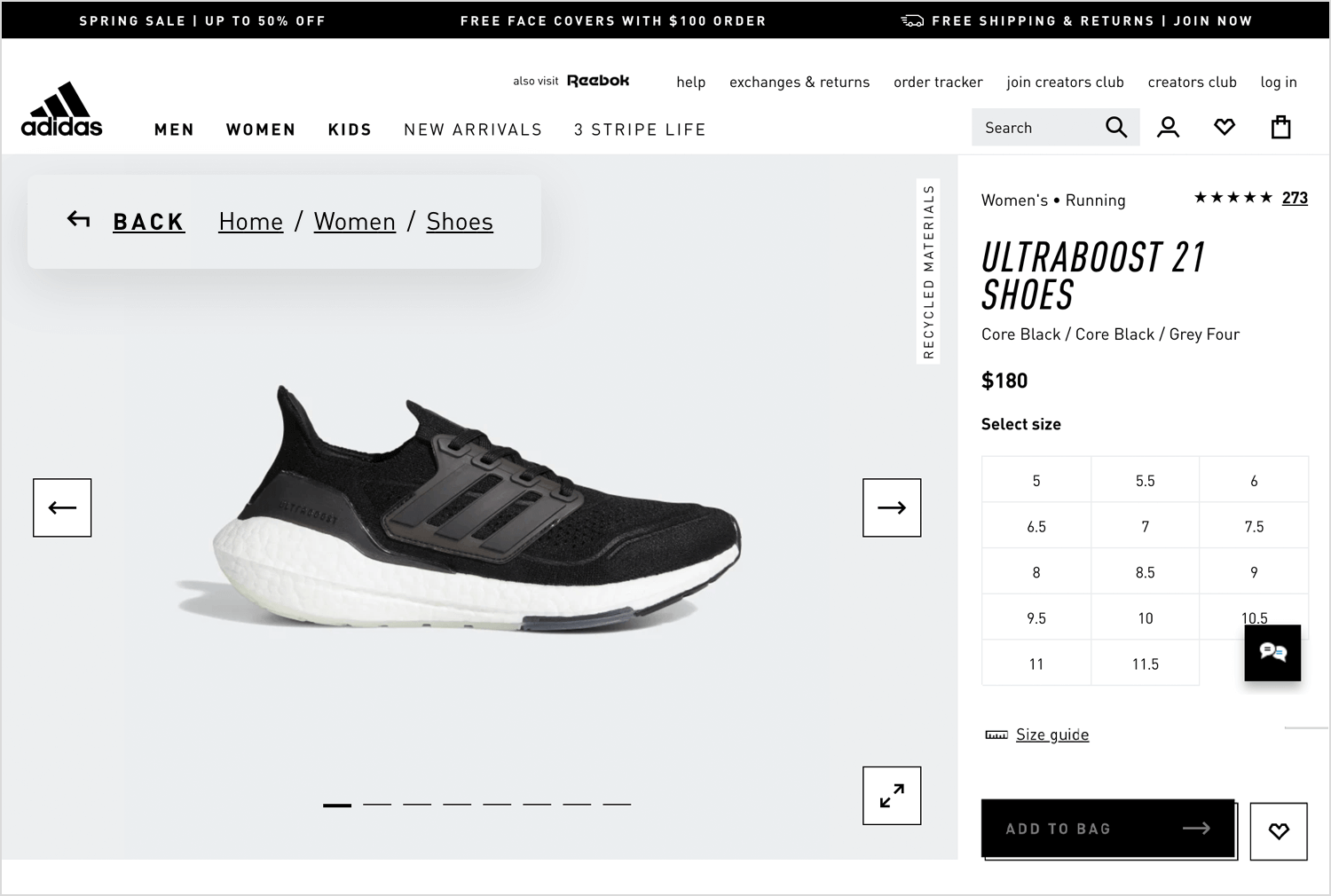This image, sourced from the Adidas website, features a detailed interface showcasing their ecommerce platform. At the very top of the page, a prominent black border displays several key promotional items: on the left side, "Spring Sale Up to 50% Off" is highlighted, while the center-right area advertises "Free Face Covers with $100 Order" and an image of a truck symbolizing "Free Shipping and Returns - Join Now." Below this black border, a white navigation bar is present, prominently featuring the Adidas logo on the left. Adjacent to the logo are category links for "Men," "Women," "Kids," "New Arrivals," and "Three Stripe Life." Just above these, user-oriented options such as "Help Exchanges and Returns," "Order Tracker," "Join Creators Club," and "Login" are available. Additionally, essential functions like a search bar, a heart icon for saved items, and a shopping bag icon are situated on the right side of the navigation bar.

The main focus of the image is located toward the bottom left, where a selected product is displayed — a sleek black running shoe with a white sole, identified as the "Ultra Boost 21 Shoes." This product falls under the "Women's Running" category and boasts a five-star rating from 275 reviews. Priced at $180, the shoe listing offers various sizes for selection and includes an "Add to Bag" button on the bottom right corner of the section, allowing users to easily proceed with their purchase.